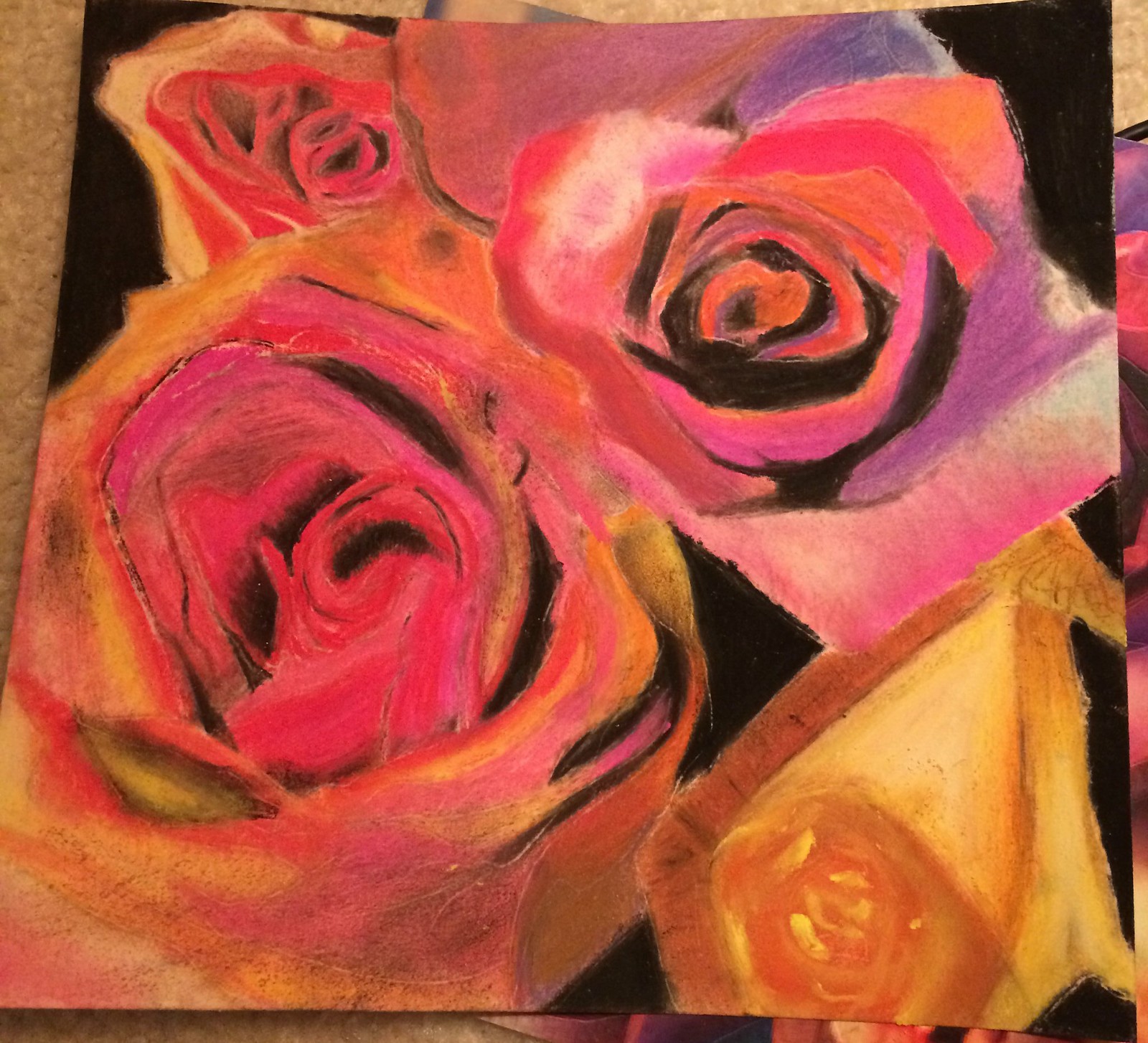This painting on canvas, possibly created with acrylics, oil paints, or pastels, showcases an impressive level of mastery over the medium. The artist demonstrates exceptional skill in the use of shadows, blacks, negative space, and color blending. The nuanced interplay of light and dark, as well as the seamless transitions between hues, reflects a high degree of technical proficiency and artistic experience that goes beyond the capabilities of an amateur.